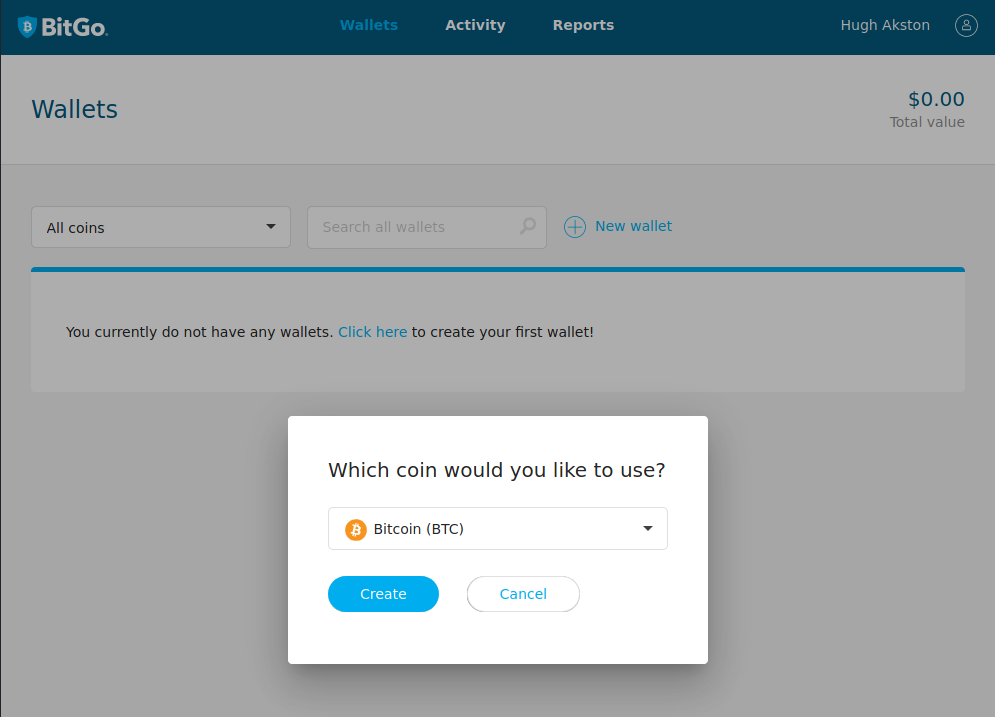Screenshot of the BitGo Website: Navigating the Wallets Section

In this screenshot of the BitGo website, the user has navigated to the "Wallets" section, as indicated by the active selection at the top of the page. The navigation bar also includes options for "Activity" and "Reports." In the upper right corner, the user is identified as "Hugh Axton," although their identity remains unknown.

Below the navigation bar, "Wallets" is highlighted in blue, indicating the current page. In the next row of options, there are boxes labeled "All Coins" with a dropdown arrow for selection, "Search All Wallets," and a circle with a plus symbol labeled "New Wallet." The "All Coins" selection is darker, signifying that it has been chosen.

A prominent blue line spans horizontally about a third of the way down the screen, displaying the message, "You currently do not have any wallets. Click here to create your first wallet." Directly below this message is a smaller white rectangle prompting, "Which coin would you like to use?" with a pre-selected option for "Bitcoin (BTC)," represented by an orange circle with a 'B' on the left side.

Toward the lower left of this section, there's a blue oval button labeled "Create," suggesting that the user is in the process of creating a new Bitcoin wallet.